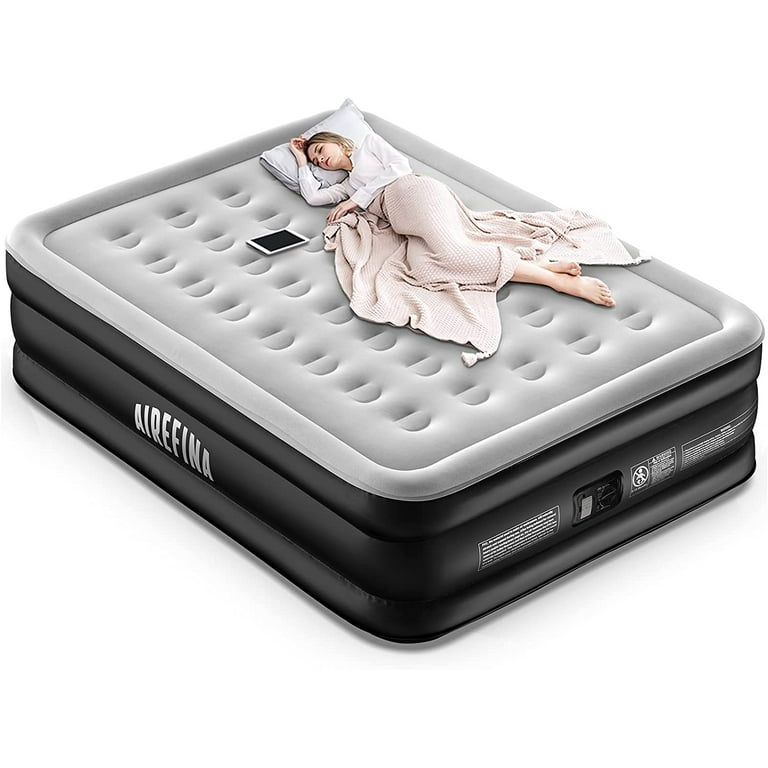A woman is relaxing on an inflatable air mattress designed for camping. The mattress has a black base with the brand name "Airefina" elegantly written in a silver arch on the side. The bottom section features a nozzle for inflation, along with visible warnings and instructions. The top surface of the mattress is light gray, covered with a fuzzy material for added comfort. The woman lies on a pillow, her arm resting by her head, wrapped in a light pink-beige blanket. Her bare feet peek out from underneath the blanket, and she is dressed in a long-sleeved white shirt. A tablet is positioned next to her, and her eyes appear open, suggesting she is awake and perhaps engrossed in her surroundings or the screen.